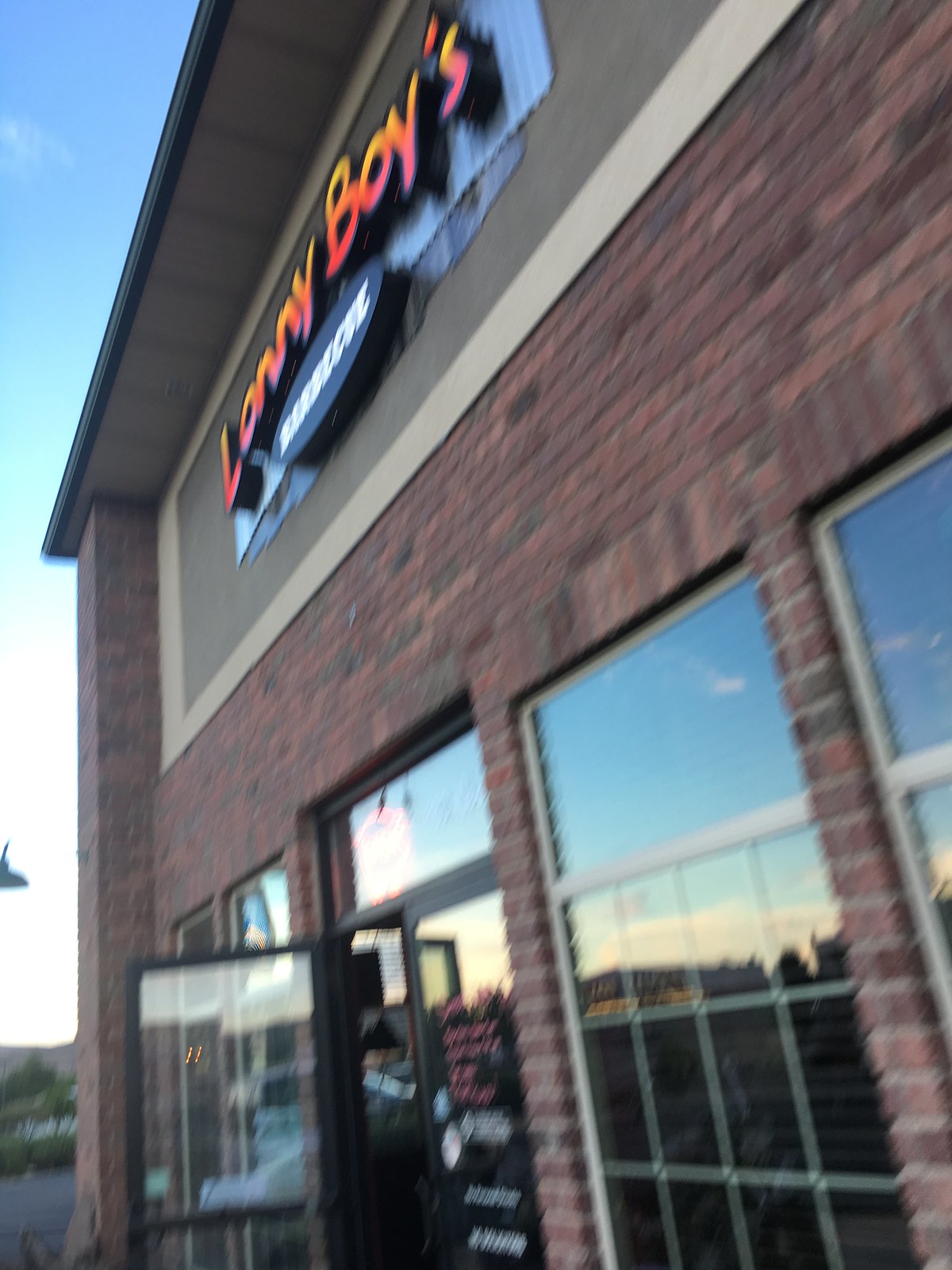This image captures the striking architectural features of a brick building from a ground-up perspective, highlighting the intricate texture and subtle hues of gray and grayish-red bricks. The backdrop is a clear, sunny blue sky that brilliantly reflects off the building's windows, adding a vibrant contrast to the otherwise muted tones of the structure. On the lower level, the reflections in the windows appear darker and indistinct, leaving their sources a mystery. The building's two glass doors draw attention; the left door stands ajar, inviting curiosity, while the right door remains closed, adorned with unreadable inscriptions. Above, under an overhang, a colorful sign catches the eye with the text "something boys" rendered in an engaging palette of orange, yellow, and pink. The first word possibly spells out "Lonny" or "Lanny," while a second, unreadable word lies beneath, adding an enigmatic touch to the scene.